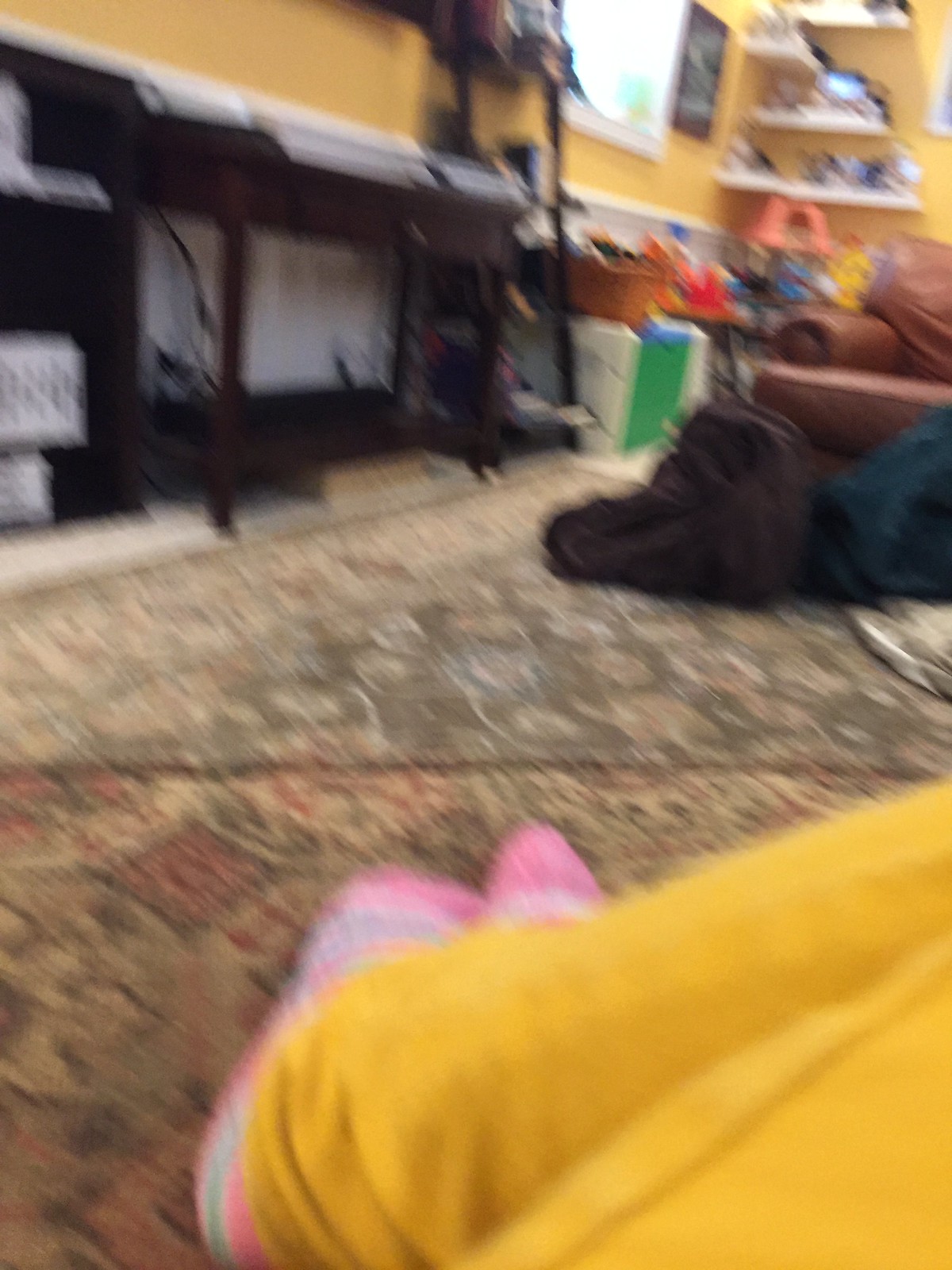This blurry, out-of-focus indoor photograph captures the view from the eye level of the photographer, seemingly taken by accident, perhaps while in motion or with a phone in a pocket. The primary focus includes the photographer's yellow sweatpants and pink, white, and teal socks. Below these, they are seated on a patterned rug that is gold and dark green with intricate floral designs, reminiscent of an oriental carpet. 

In the background against a mustard yellow wall, the scene details a white trim separating the upper and lower sections of the wall. There is a white shelf running parallel to the wall, and alongside it are three more white shelves that contain what appear to be children's toys. A small, framed picture sits next to a square-shaped window emitting light. Below the shelves stands a brown leather couch, with a black and a green blanket balled up on the floor in front of it. To the left, a table and a TV stand are positioned, contributing further to the lived-in ambiance of the room.